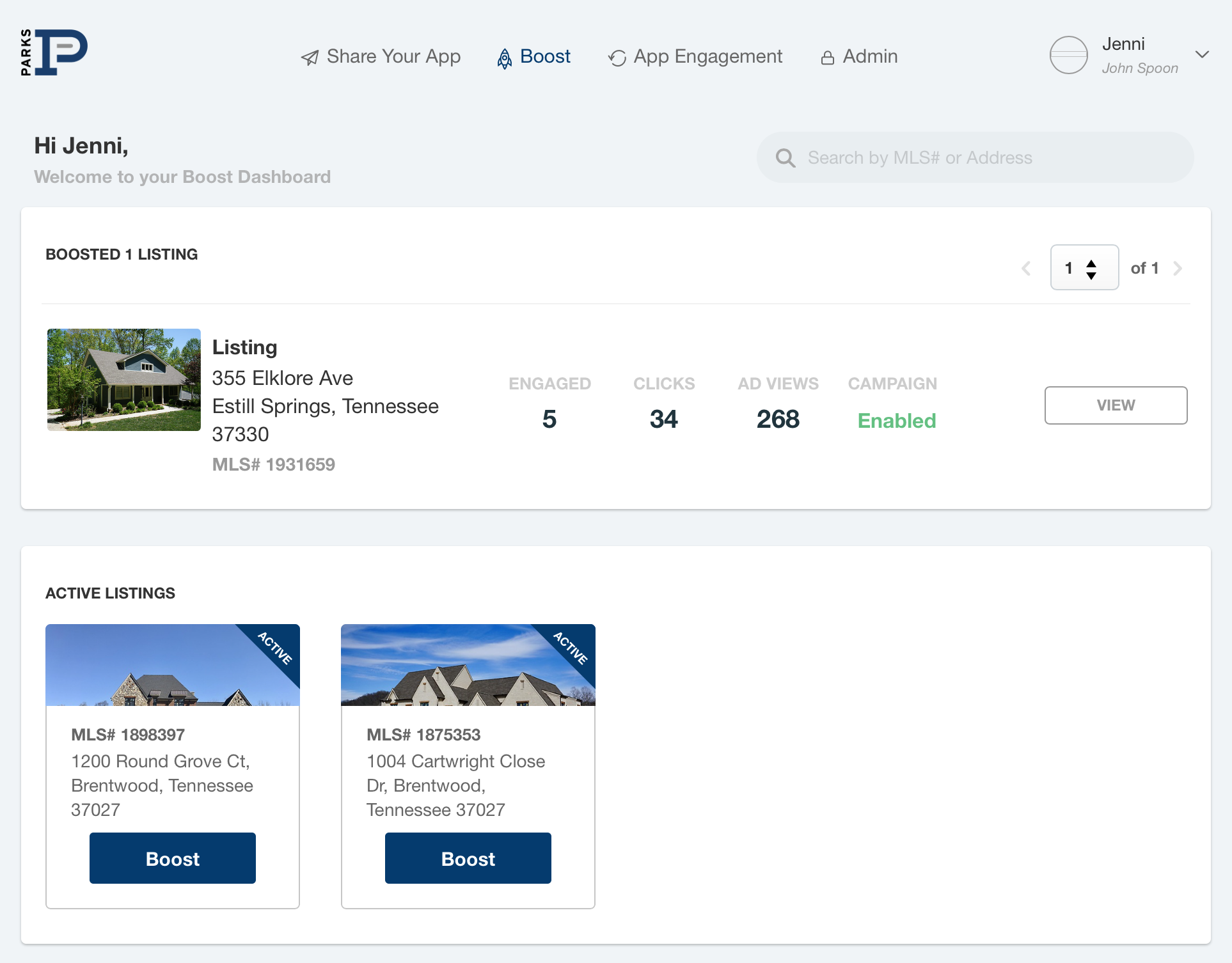The image features a light gray and white interface with detailed sections of information. 

At the top section, the background is predominantly light gray, interspersed with two white sections. In the top left corner, there is a Parks logo, which consists of a capital "P" in blue with a gray dash in the middle. The word "Parks" is written vertically to the left of the "P" in black. To the right of the Parks logo, there is text in gray reading "Share Your App". Further to the right, the word "Boost" is highlighted in blue, followed by "App Engagement" and "Admin" both in gray. The name "Jenny" (J-E-N-N-I) appears in gray as the account name, with "John Spoon" written underneath in a lighter gray. A gray circle to the left of the name displays two horizontal light gray lines across its center. 

Beneath this top section, there’s a greeting in black text: "Hi Jenny" followed by "Welcome to your Boost Dashboard". To the right of this greeting, there is a gray search bar and search icon. 

The middle section features a white rectangle that reads "Boosted 1 Listing" with an image of a house to its left. Following the image, detailed text includes:
- Listing: 355 Elkhorn Avenue
- Estill Springs, Tennessee
- 37330
- MLS number

To the right of the property details, there are metrics displayed in a vertical format:
- "Engaged" in gray with the number "5" in black underneath
- "Clicks" in gray with the number "34" in black underneath
- "Ad Views" in gray with the number "268" underneath
- "Campaign" in gray with the status "Enabled" in green underneath

Adjacent to this section is a white rectangle labeled "View" in gray text.

The next section below displays "Active Listings" in black font. There are two images of houses partially visible, showing only the sky in the background—one with blue skies and another with clouds. Each of these listings has an address and MLS number below them. At the bottom of each listing, a navy blue rectangle with white text reads "Boost".

Each element in the image has been meticulously detailed to provide a comprehensive understanding of the interface and its contents.